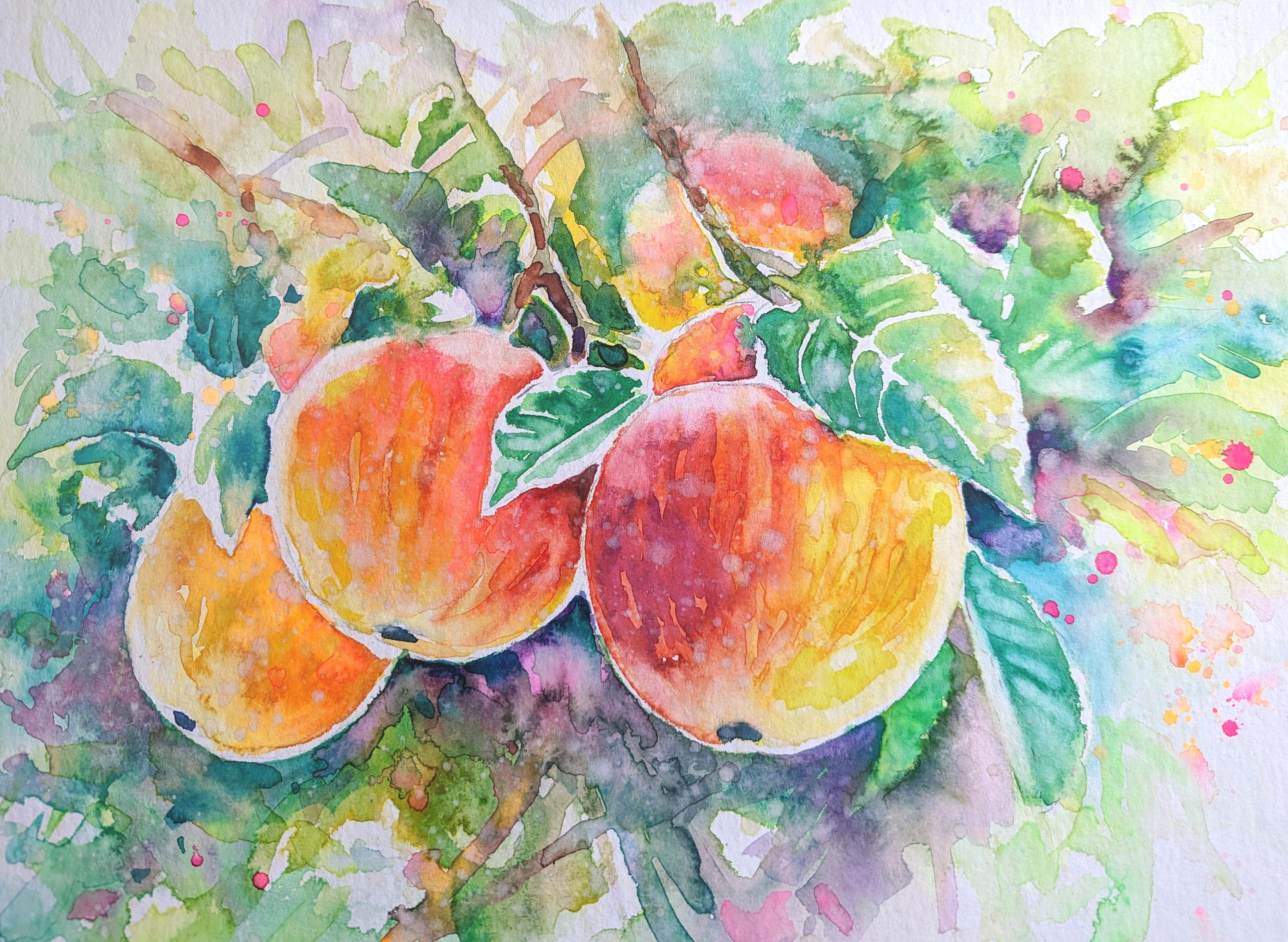This vibrant watercolor painting depicts a fruit tree, likely a peach or apple tree, with an emphasis on its contemporary artistry. Four pieces of fruit, predominantly in hues of orange and red suggesting ripened stages, hang from the branches. The fruits are accentuated with pastel colors, deviating from typical fruit shades, making their identification challenging. The leaves, meticulously detailed with veins, showcase an array of colors including greens, reds, pinks, yellows, and purples, enhancing the overall whimsical nature of the piece. The tree branches are a subtle brown, providing a natural contrast. The background, a blend of muted, splattered watercolor shades of green and yellow, serves to bring focus to the central elements – the fruits and leaves. This artwork masterfully presents a contemporary spin on a traditional still life, encapsulating the beauty through a blend of detailed elements and abstract splatters.